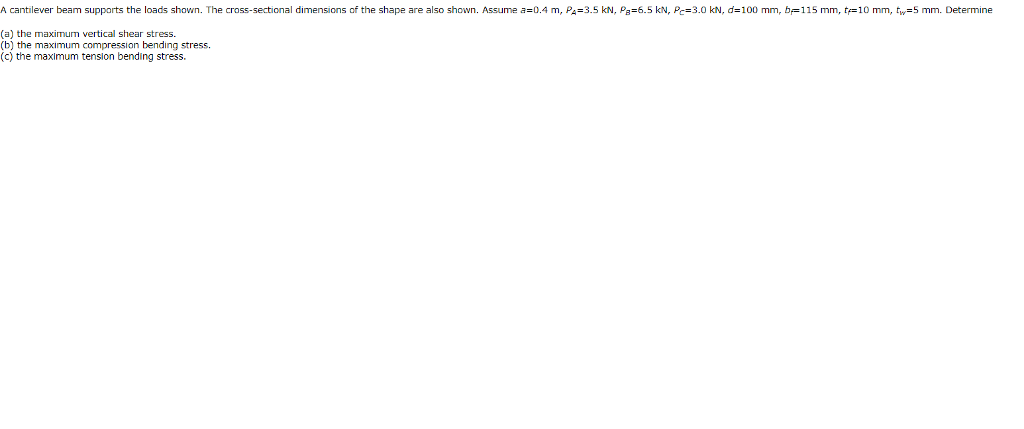This image shows a screenshot with black text on a white background, occupying the entire top portion of the image. The text is organized in a detailed manner, presenting a problem involving a cantilever beam. The word "cantilever" is prominently displayed at the beginning, spelled out as C-A-N-T-I-L-E-V-E-R.

The caption provides the following information:

"A cantilever beam supports the loads shown. The cross-sectional dimensions of the shape are also shown. 

Assume:
- A = 0.4 M
- PA = 3.5 KN
- PB = 6.5 KN
- PC = 3.0 KN
- D = 100 mm
- B = 115 mm
- T = 10 mm
- TW = 5 mm

Determine:
A. The maximum vertical shear stress.
B. The maximum compression bending stress.
C. The maximum tension bending stress."

The text is precise, indicating specific physical dimensions and loads applied to the cantilever beam, and it prompts the reader to determine the maximum stresses in various scenarios.